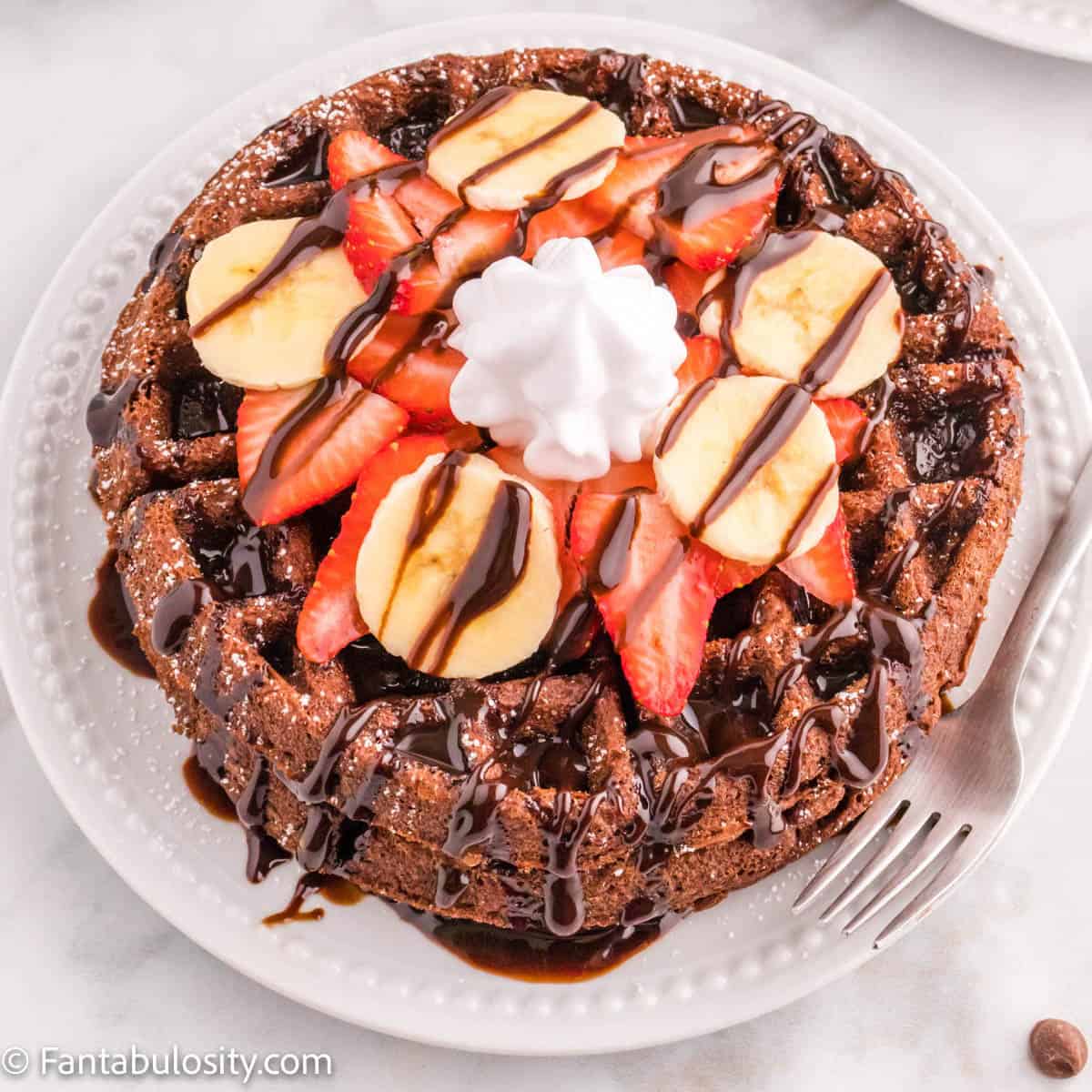The image captures a delectable dessert of two round, deep brown waffles stacked atop one another on a white plate adorned with white dots around the edge. The waffles are topped with fresh, sliced strawberries and five slices of banana, and a single dollop of whipped cream sits at the center. Rich chocolate sauce is drizzled generously over the waffles and fruit, with some of it spilling over the sides onto the plate. To the bottom right, a silver fork rests, tines down, on the plate. The setting appears to be a white tablecloth, and in the bottom left corner of the image, the text "FantaBoloCity.com" is visible, indicating a possible source or copyright.